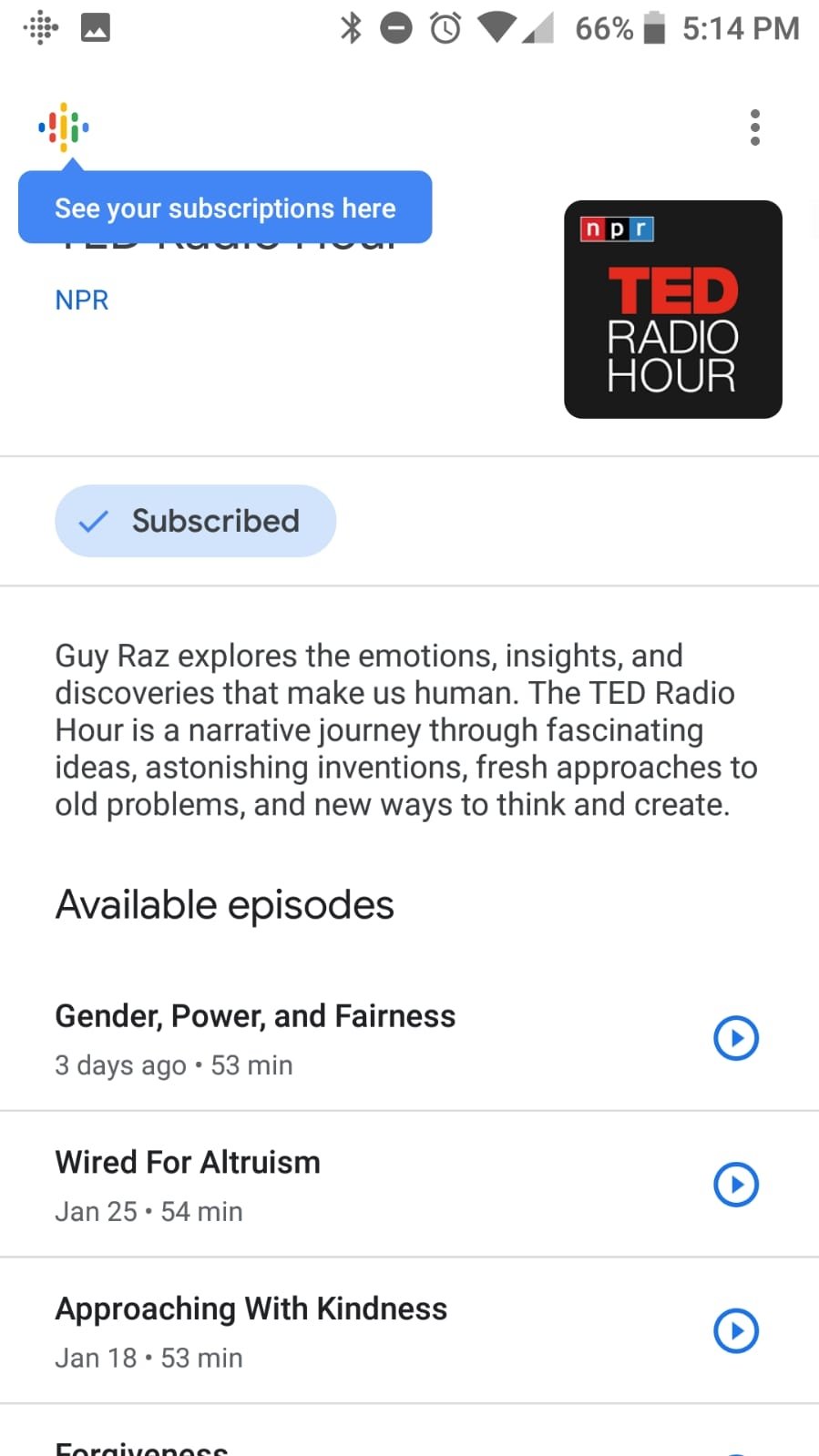This image is a screenshot of a cell phone screen displaying an NPR Ted Radio Hour podcast interface, set against a white background that seamlessly blends in. The top section reveals a typical smartphone status bar featuring multiple icons: two on the left and seven on the right. These icons include an alarm clock, a Bluetooth symbol, and a battery indicator showing 66% charge. The current time is displayed as 5:14 p.m.

In the upper left-hand corner, there is a diamond-shaped icon adorned in Google’s characteristic colors, accompanied by a blue tooltip that reads in white text, "See your subscriptions here." Adjacent to this, on the right, there's a rounded-corner square with a black background showcasing the NPR Ted Radio Hour logo. A blue oval button labeled "Subscribed" is visible just below the logo.

Below this, the screen lists available episodes of the podcast, each accompanied by a brief description. The episodes shown are:

1. "Gender, Power, and Fairness," released three days ago, lasting 53 minutes.
2. "Wired for Altruism," dated January 25th and lasting 54 minutes.
3. "Approaching with Kindness," dated January 18th and lasting 53 minutes.

Further down the page, there are additional episodes, partially visible, with one appearing to have the word "forgiveness" in the title. Scrolling down would reveal the complete list of episodes.